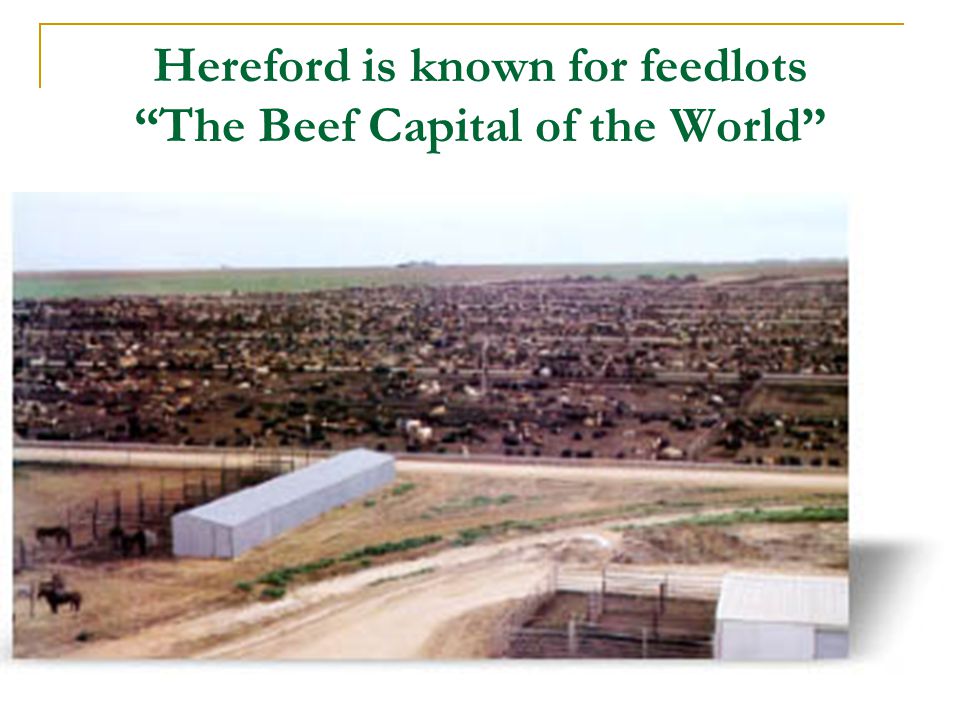This aerial color photograph showcases a vast cattle ranch under a vivid blue sky. A bold gold line runs across the top of the image, accentuating green text that declares, "Hereford is known for feedlots (the beef capital of the world)." The expansive ranch below features a long, rectangular silver shed on the bottom left, beside a dirt path winding horizontally across the image. Green bushes speckle the foreground near another dirt area, potentially a road, which intersects with a vertical dirt path starting at the bottom left and extending to the middle right. On the bottom right corner, a wooden-fenced pen houses a partially visible shed. Scattered across the landscape are various buildings and large, brown fields, where clusters of cattle and other livestock graze nearby. The image captures a mixture of green grass, dirt, and sprawling feedlots, affirming Hereford's reputation in the beef industry.